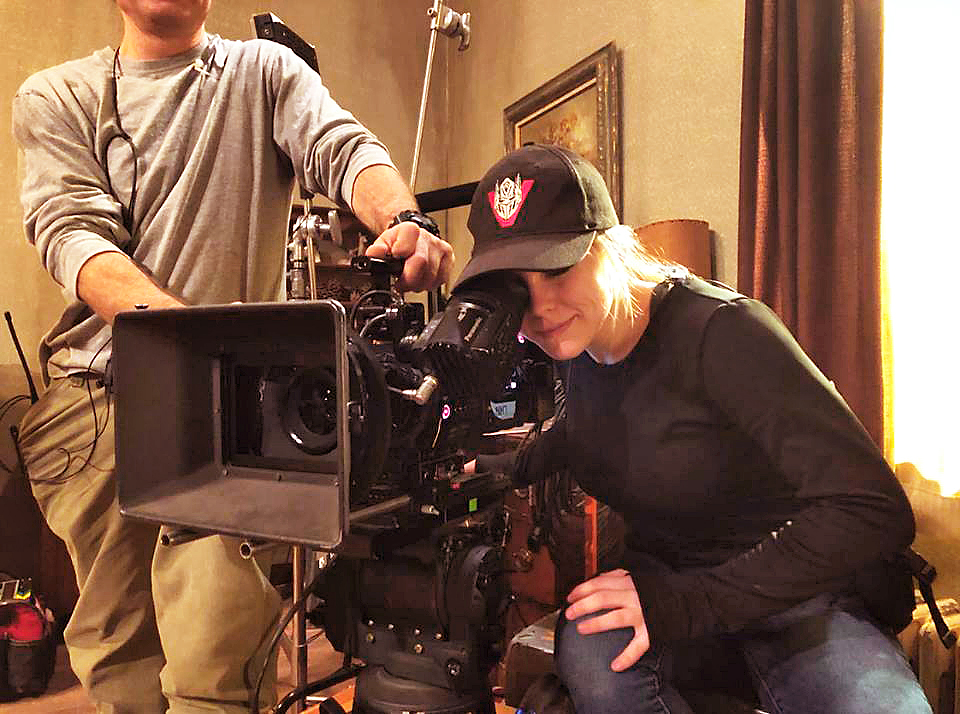In the image, a woman is seated in a room with brown accents, including brown curtains, cream-colored walls, and framed wall art. She is looking through the viewfinder of a professional-grade video camera. She is wearing a black long-sleeved shirt, a pair of light blue jeans, and a black baseball cap adorned with a logo featuring a skull and a red triangle, or possibly a transformer logo. Her blonde hair is tucked under the cap, and her right eye is pressed up against the camera's viewfinder. Beside her, on the right side of the frame, stands a man whose head is cut out of the image. He is dressed in a gray, round-neck long-sleeved sweater with the sleeves pushed up to his elbows, and tan khaki pants. The camera, black in color, is equipped with numerous switches and knobs. Overall, the scene suggests a professional or film set environment with sunlight streaming through a window, enhancing the room's warm tones.